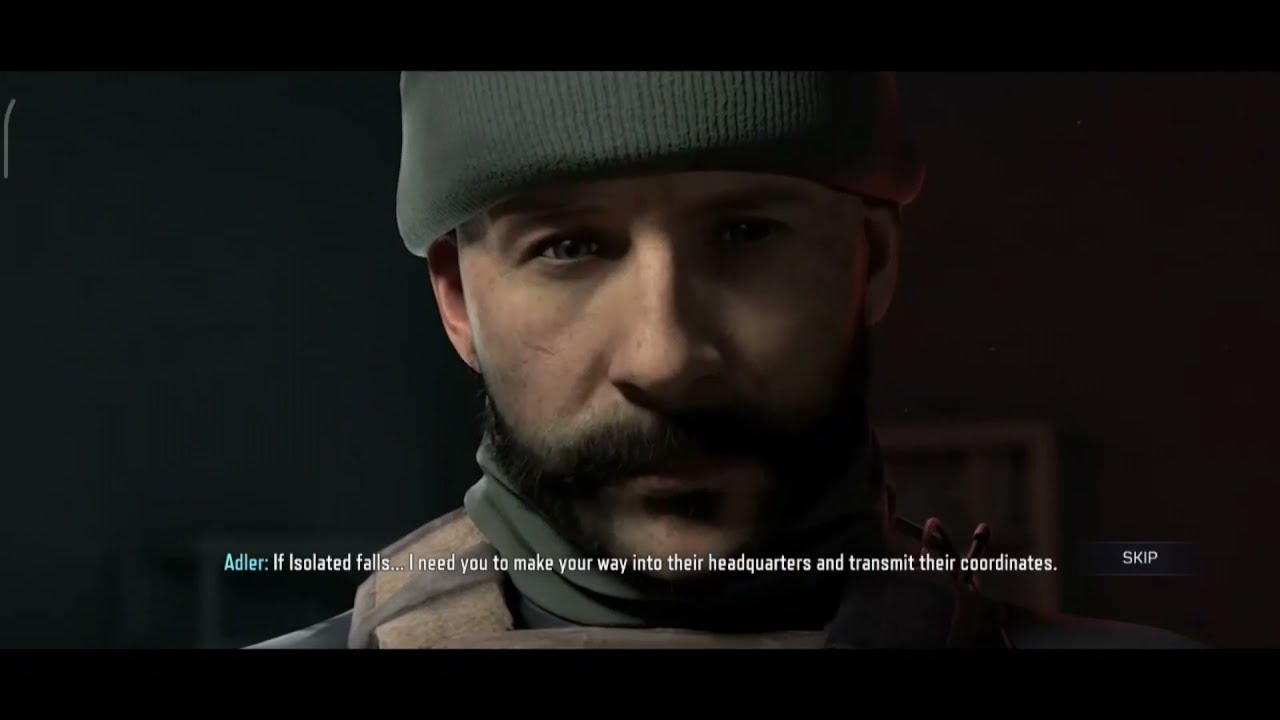The image is a highly detailed screenshot from a new generation video game, likely from the Call of Duty series, indicated by the graphical quality suggestive of a PS5, new Xbox console, or high-end PC. It features a close-up of a middle-aged white man with a brown goatee and beard, wearing a green beanie resembling an army hat and a turtleneck. He is staring directly into the camera, and behind him is part of a wall and a picture frame. The image appears to be from a cutscene, as evidenced by the presence of subtitles in the scene. The text reads, "Adler: If isolated falls, I need you to make your way into their headquarters and transmit their coordinates," with "Adler" in blue font and the rest in white. Additionally, there is a "Skip" button in white font within a small dark gray box, allowing players to bypass the cutscene. The scene is framed by black horizontal bars at the top and bottom, focusing attention on the central visual and narrative elements.